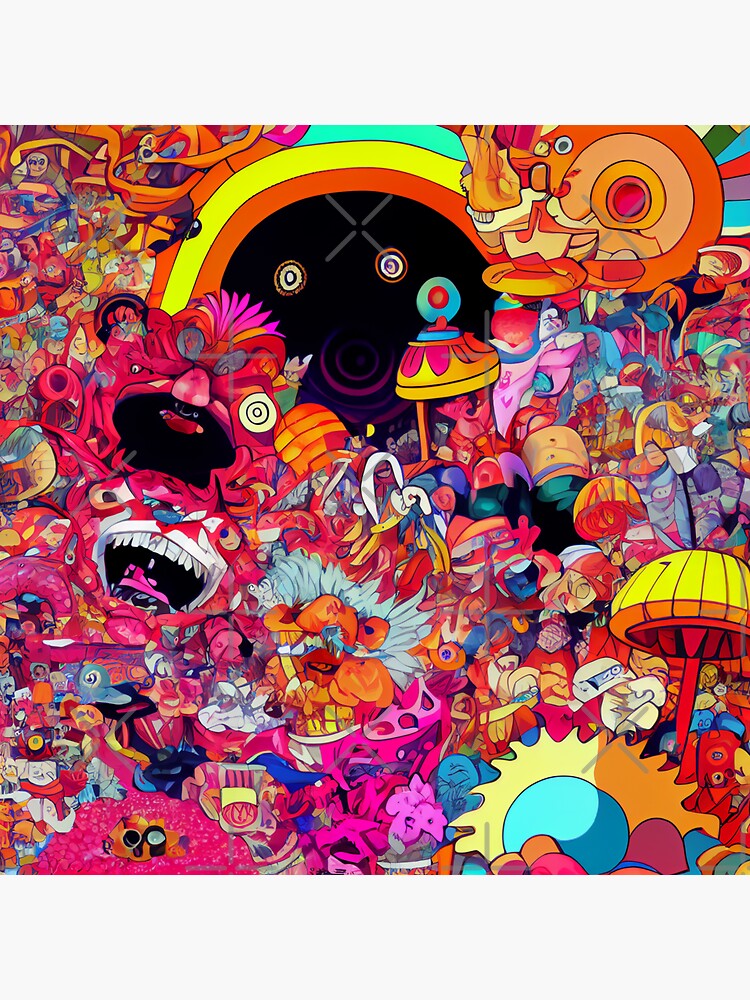This vibrant and wild image presents a chaotic, colorful scene that feels both cartoon-like and somewhat eerie. Dominating the top center is a large, black smiley face, encircled by a rainbow of green, yellow, and red hues. Throughout the picture, a crowd of abstract, brightly-colored figures and monster-like critters with black faces and sharp white teeth can be seen, adding to the bizarre atmosphere. On the left side, a large creature resembling a dog grins menacingly, showcasing its sizable, open mouth and numerous teeth. The bottom right corner features mushroom shapes and an upside-down cup colored yellow and red. Additionally, there’s a noticeable orange circle with a pink center in the top right, adorned with multicolored feathers extending from one side. The composition is a mesh of various forms and colors, predominantly pink, blue, yellow, red, and green, creating an engaging visual experience that is equal parts playful and unsettling.